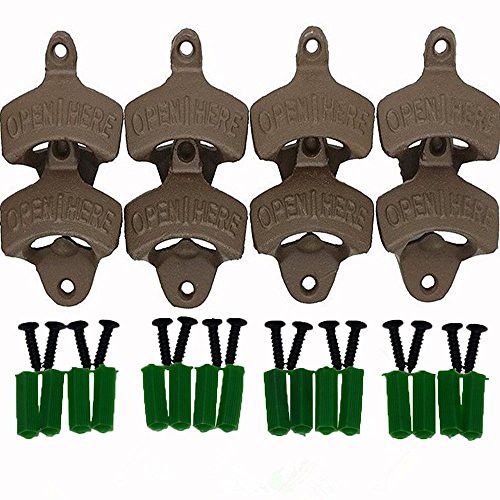This is a detailed photograph of eight wall-mounted, pewter-colored metal bottle openers arranged in two rows of four against a stark white background. Each bottle opener features raised lettering that reads "OPEN HERE," split between the 'N' and the 'H' by a single vertical raised line. The top of each opener has a small spike with a hole, suggesting it can be hung, and the bottom features a curved section with another hole, providing additional support when mounted. Below the bottle openers, there are 16 green drywall pegs and 16 brown screws neatly organized for securing the openers to the wall. The overall scene presents a clean, methodical layout with the practical accessories prominently displayed beneath the bottle openers.